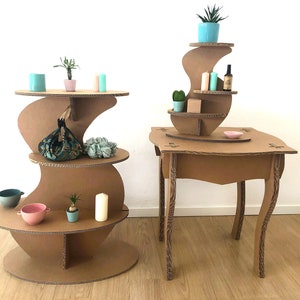The image features two distinct pieces of eclectic brown furniture set against a white wall with narrow white molding and a light-colored hardwood floor. On the left side, there's a unique multi-tiered table with three circular shelves, supported by an S-shaped panel that winds through all three levels. The shelves are adorned with various knickknacks including bowls, candles, rocky or flowery designs, and small plants. To the right, there's a square wooden end table with slightly curved legs that taper down to the ground, complemented by a front bar supporting the tabletop. This end table also has a miniature version of the multi-tiered table placed on its top, similarly decorated with small plants, candles, and a bottle. The photograph is clear and brightly lit, highlighting the details of the furniture and the arrangement of items on them.